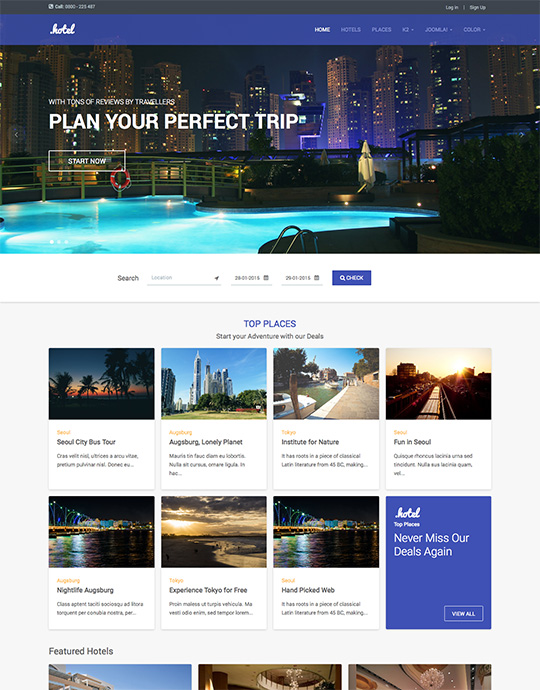The image features a website interface with a predominantly black background and white text in the upper left corner, displaying an unreadable phone number due to its small size. On the right side, the options to "Log In" and "Sign In" are clearly visible. Below, against a very dark blue background, the word "Hotel," written in cursive white text, stands out. To the right, there is a navigation menu with "Home" in white text, followed by grey text listing options such as "Hotels," "Places," and other unclear categories.

The backdrop includes a striking city skyline, captured at night, with towering skyscrapers illuminated by yellow lights. On the left, white text reads, "With tons of reviews by travelers, plan your perfect trip." Below this, a button labeled "Start Now" is prominently displayed. Underneath lies a white search bar bordered by black text indicating "Search." This section allows users to input their location and select start and end dates. Adjacent to these fields, a blue box with white text prompts users to "Check for your dates."

Further down, a grey background features a title in blue text, "Top Places," followed by the tagline in grey, "Start your adventure with our deals." Seven clickable destinations are listed, including "Seoul City Bus Tour," "Augusta Lonely Planner," and "Fun in Seoul." These options suggest various attractions and experiences in South Korea.